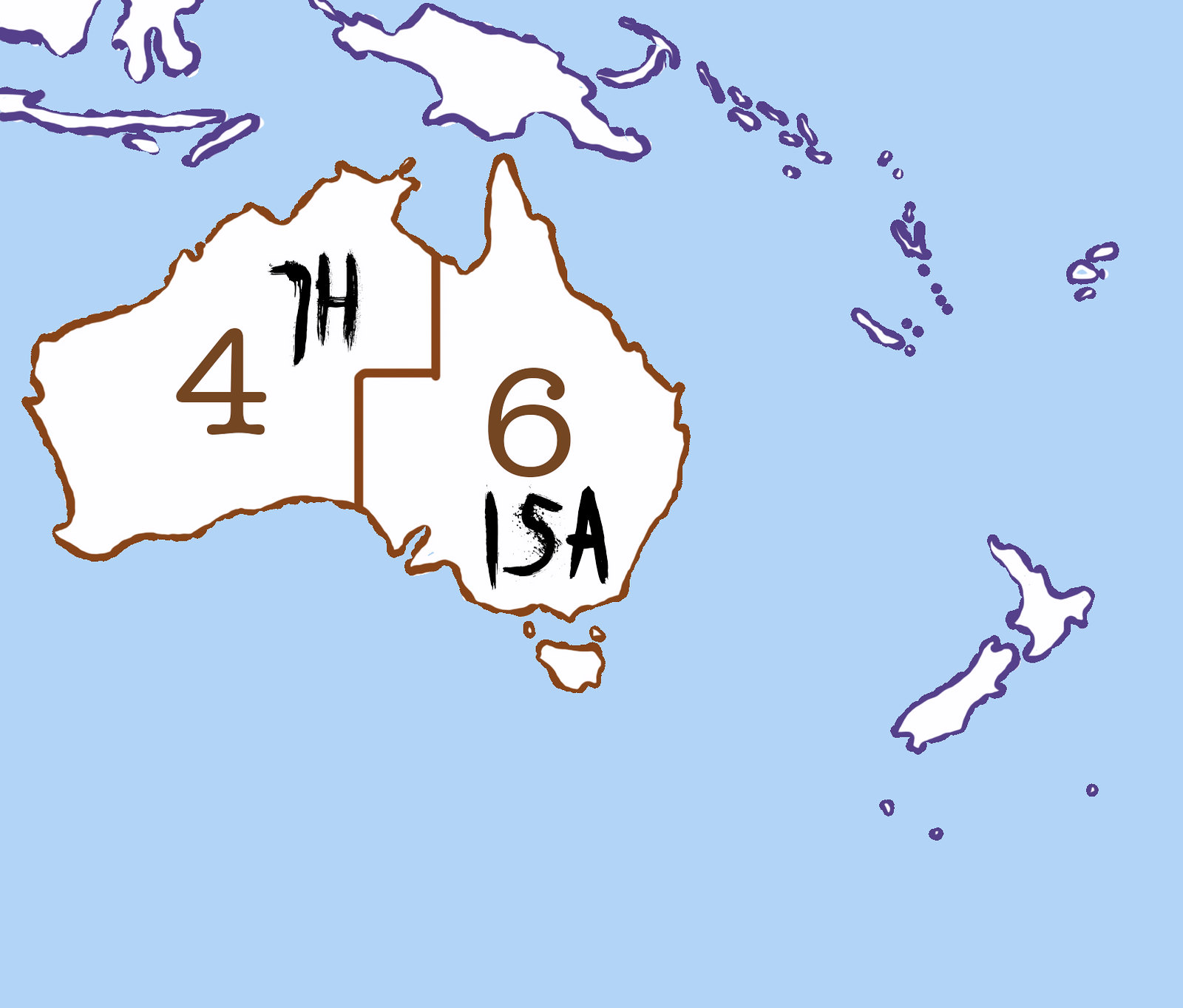This is a slightly wide rectangular digital image of a close-up map with a light blue background resembling water. In the top left corner, several small white blobs surrounded by purple and blue outlines represent island clusters, extending towards the center and then downwards. Centrally on the left, a prominent angular landmass, evocative of Australia, is bordered in brown with an off-white interior. This larger island is divided by a brown line that zigzags left and right, with the left section marked by "4" and "7H" in brown and black ink respectively, while the right section bears the numbers "6" and "15A" in brown. Nearby, towards the bottom right corner, lies another white island outlined in purple, accompanied by a scatter of smaller white islands with blue and purple borders.